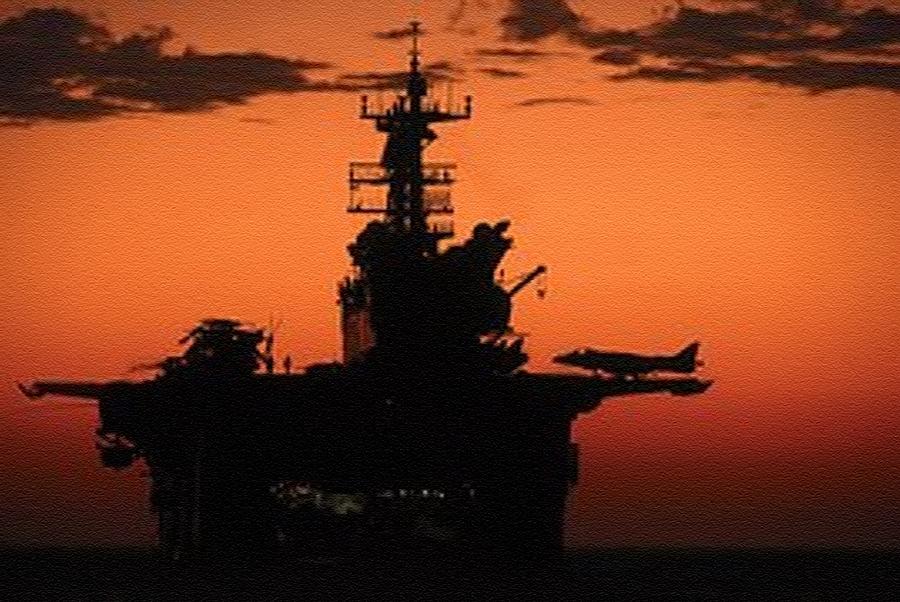The image captures a dramatic maritime scene at either sunset or sunrise, casting an orangish-yellow hue across the sky that transitions to a darker shade near the horizon. Wispy, dark gray clouds drift across the scene, partially silhouetted by the fading sunlight. A large naval ship dominates the view, its silhouette sharply outlined against the glowing sky. The ship features a prominent tower just right of the center, topped with what appears to be a radar screen. On the deck, there is a distinct, flat surface that serves as a landing area for aircraft. To the right, a plane is visible, oriented towards the ship's center. On the left side of the deck, another aircraft, possibly a helicopter, is discernible despite the shadows, with empty space extending to the ship's edge. The ship's bulk extends down into the water, rendered in dark silhouette against the lighter horizon. The bottom of the image is shrouded in darkness, where the water merges indistinctly with the edges of the vessel and the surrounding environment, completing the somber, majestic scene.